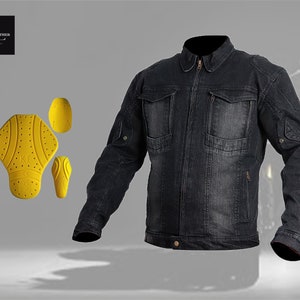The image appears to be an advertisement set against a plain white background, featuring a large, black denim jacket positioned as if worn, though no person is inside it. The jacket, which takes up approximately three-quarters of the picture, has a rugged look with fading, chest pockets, side pockets, and sleeve snaps. It zips up the front and has a snap at the waistband, giving it the appearance of motorcycle fashion.

To the left of the jacket are three yellow objects, resembling elements of a bicycle seat or possibly parts of an insert for shoes. These objects have distinctive shapes: holes and lines similar to a baseball pattern mark the main, larger piece, which is wide at the top and narrows toward the bottom. Two smaller, similar yellow pieces complete the arrangement. Additionally, there is a partial text box cut off along the left edge of the photo, suggesting this is promotional material. Shadows beneath the jacket emphasize its three-dimensional form.